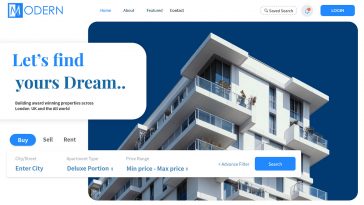The image features a modern white apartment or condominium building set against a deep blue sky, suggesting a serene, clear day. Captured from a low angle, the photograph draws the eye upward along the structure’s clean lines, emphasizing its height and architectural design.

Prominently displayed on the building façade is the branding of a company called Modern, with their name in blue. The distinctive logo features a stylized "M" within a square that is half blue and half white. 

At the top of the image, there are small keys depicted, though they are somewhat difficult to discern. Below this section, a clickable blue button invites users to "Let's find your dream," encased in a white speech bubble, indicating a call to action for prospective clients. Beneath this, there is a segmented blue bar with options for "Buy," "Sell," and "Rent," each in white text, directing users to the respective services they seek.

Further down, a search bar is provided where users can enter their city. The fine print offering additional options appears too small to be easily readable. On the right side of the search bar, there is another blue button designated for submitting personal information.

Overall, this image not only highlights the sleek design of the residential building but also engages potential clients with clear, interactive elements to assist in their search for real estate services.